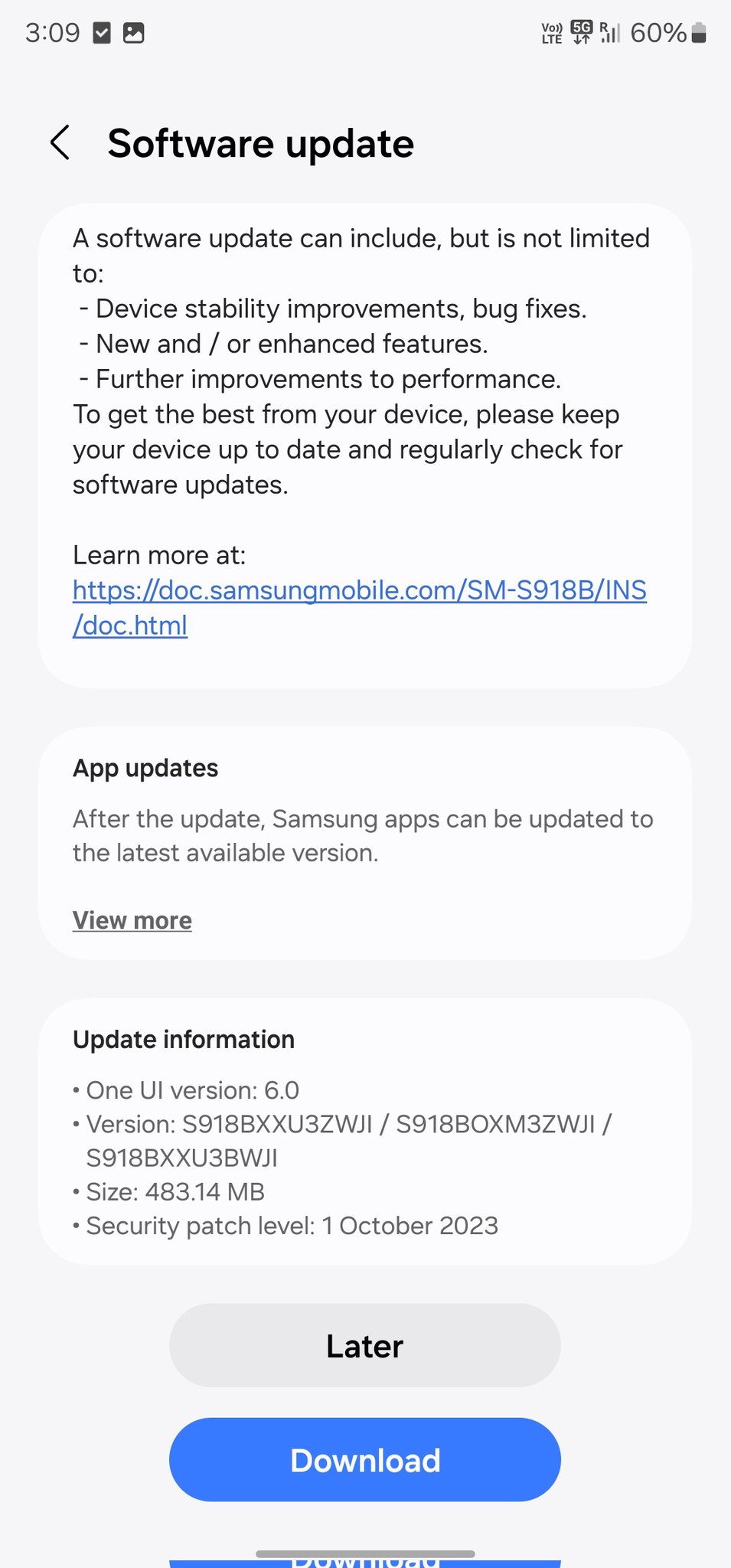**Caption:**

In this vertically-oriented rectangular image, which appears to be a screenshot from a smartphone, a concise overview of a software update is displayed against a light gray background. The image captures the top section of the phone screen, where the current time, 3:09, is shown in the top left corner. Two unidentified icons are positioned next to the time. On the top right, several status indicators are visible, including a 5G symbol, a cellular signal strength indicator showing three or four bars, a battery level at 60%, and a battery icon.

Prominently displayed in bold black text is the heading "Software Update," accompanied by a rightward-pointing arrow. Below this, in a white text box, detailed information about the software update is provided, emphasizing possible improvements such as device stability, bug fixes, new or enhanced features, and performance enhancements. The text encourages users to keep their devices up to date for optimal performance with a note to regularly check for updates. A blue-underlined hyperlink, which reads "Learn more at https://doc.samsungmobile.com/SMSN18B/INS/DOC.html," provides additional details.

Further down, a section titled "App Updates" indicates that Samsung apps can be updated to their latest versions following the software update. A "View more" option is available to explore additional information.